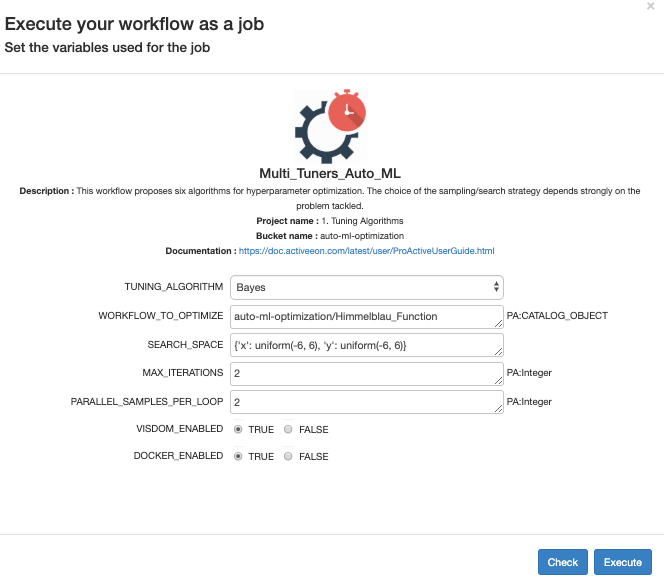**Detailed Caption:**  
The image showcases a section of a web-based interface related to job execution within workflow management. In the top-left corner, the heading "Execute your workflow as a job" indicates the primary focus of the platform being displayed. Directly below this heading, the text instructs users to "Set the variables used for the job."

On the top-right side of the image, a subtle 'X' icon in light grey can be seen, likely serving as a close or exit button for the current view or pop-up.

Centrally positioned towards the top, albeit slightly lower than the topmost text, there is a gear icon with a red clock icon overlaying its top-right corner, suggesting settings related to time or scheduling. Adjacent to this icon, the label reads "Multi-Tuners Auto ML," highlighting an automated machine learning feature involving multiple tuners.

Beneath this, on the left-hand side, there is a section starting with the label "Description:" followed by a detailed explanation: "This workflow proposes six algorithms for hyper-parameter optimization. The choice of the sampling search strategy depends strongly on the problem tackled."

Further down, the "Project Name: Tuning Algorithms," followed by "Bucket Name: Auto ML Optimization," indicates specific project and storage identifiers. There is also a mention of "Documentation" with an accompanying hyperlink, suggesting the availability of further reading or instructions.

Directly below, several text boxes are aligned vertically. The first text box contains the word "Bayes" under the label "Tuning Algorithm." Four additional text boxes follow in subsequent rows, although their contents are not described.

In the bottom-left corner of the image, there is an option labeled "Wisdom Enabled," with a toggle indicating that the 'True' option is selected while the 'False' option remains unselected. This likely pertains to a feature or mode within the platform.

Overall, the image captures a sophisticated interface designed for configuring and optimizing workflows through algorithm selection and detailed parameter settings.